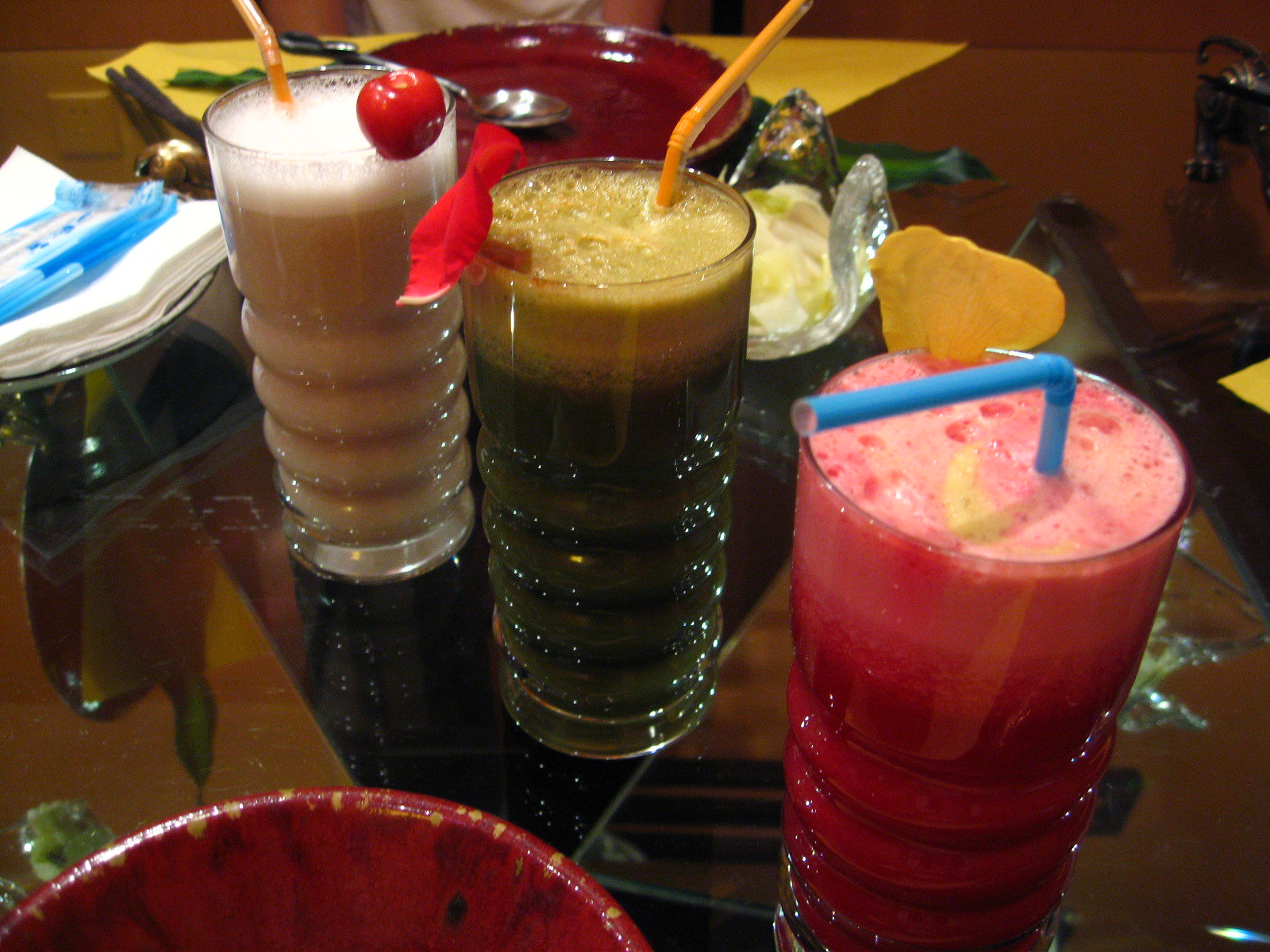This vibrant and colorful photograph showcases three ice cream sodas arranged diagonally on a reflective glass tabletop, likely in a restaurant setting. The drinks are presented in textured translucent glasses, featuring ribbed patterns that transition to smooth near the top. Each glass captures the bright overhead lights, adding a dynamic gleam to the scene. The frontmost soda, located at the bottom right, is a strawberry-flavored drink with a reddish-pink hue topped with pink foam and a blue straw, adorned with some ornamentation. Positioned centrally is a green-hued soda with foam, possibly a root beer float, featuring an orange straw. In the background, the third drink is a light brown concoction, resembling a chocolate cream soda, capped with white foam and garnished with a cherry on the rim. The artistic arrangement and the vibrant colors of the surrounding elements contribute to an enticing and appetizing visual experience.